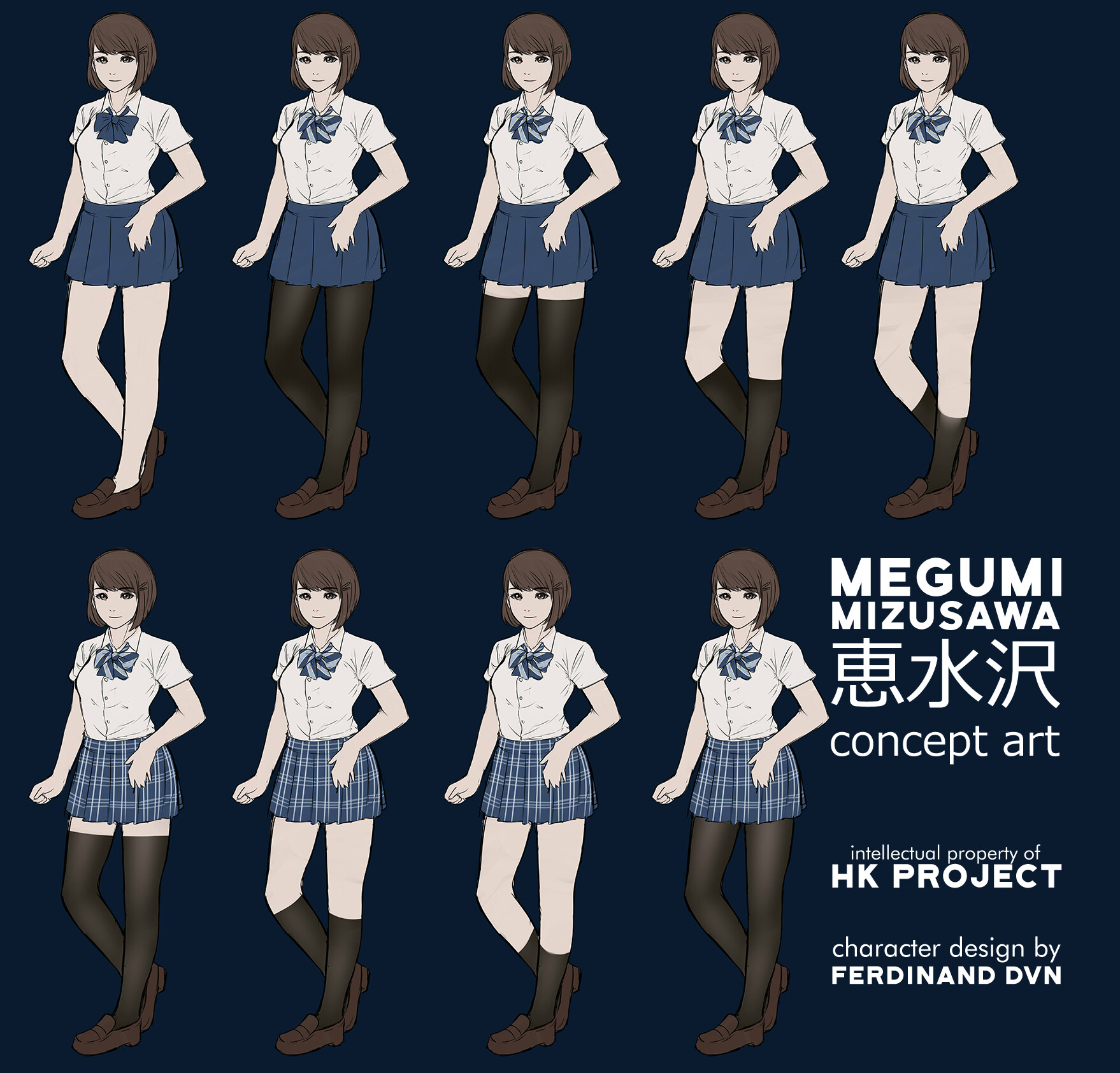This image appears to be a detailed concept art poster for character design, showcasing variations in legwear for a female anime character named Megumi Mizusawa, intellectual property of the HK Project. The character, designed by Ferdinand DVN, is depicted in nine different illustrations. She is consistently dressed in a school uniform featuring a button-up shirt, a blue skirt, and brown loafers. Her short brown hair is styled in a bob, and she has a blue bow tie. 

In the different illustrations, her legwear varies significantly. Some variations include very long thigh-high socks, knee-length socks, and mid-shin socks, while in a few images she isn't wearing any socks at all. Additionally, the tights and socks shown are mostly black. The top row of images shows her in a plain blue skirt, while in the bottom row, she wears a blue and white checkered skirt. This poster not only highlights different types and lengths of socks and pantyhose but also emphasizes subtle changes in the character's appearance to showcase the versatility and detail in her design.